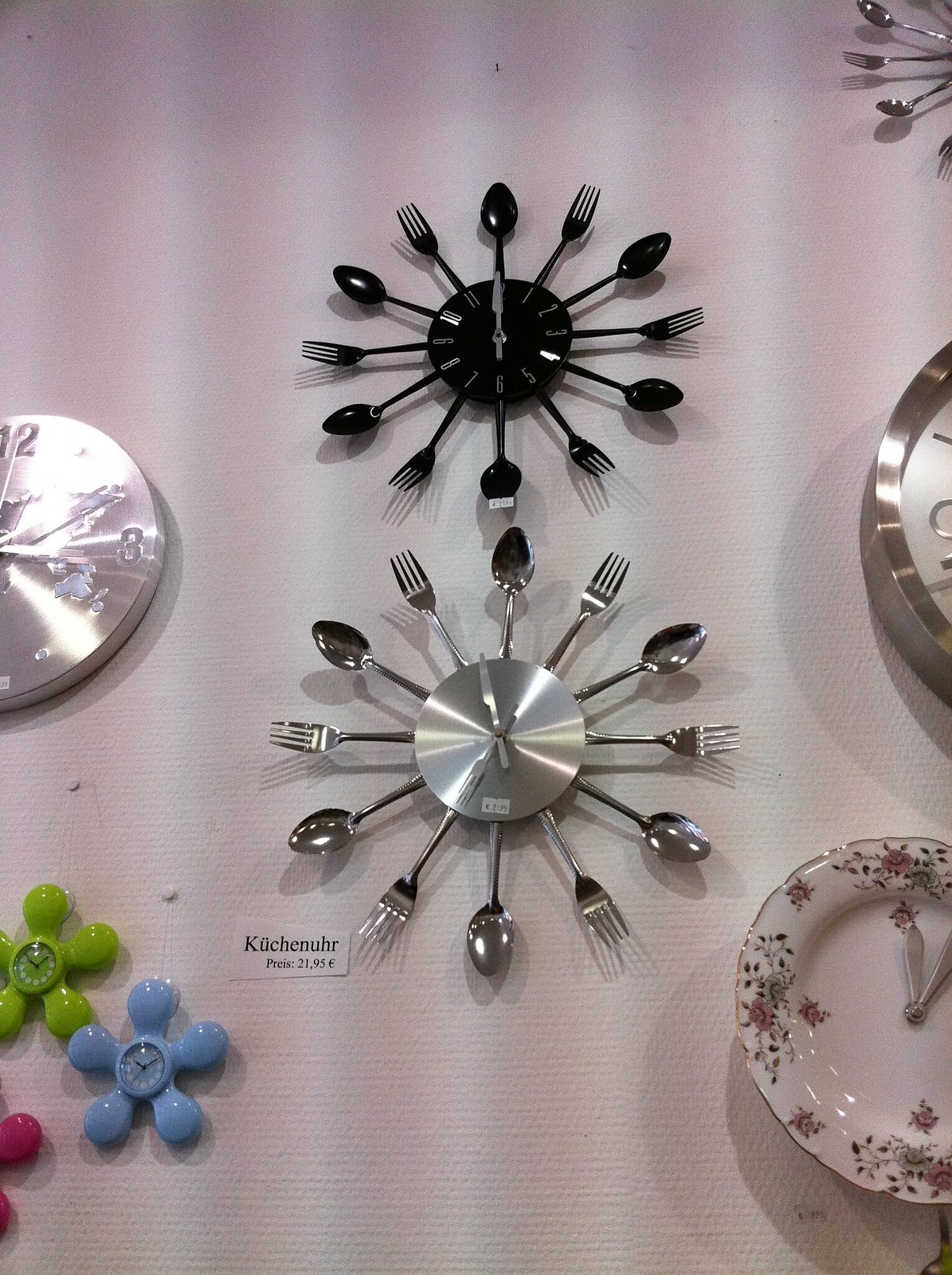The photograph showcases an artistic display of two creatively made clocks set against a slightly pinkish white or embossed tablecloth backdrop. Central to the image, positioned vertically, are two elaborately designed clocks, each using cutlery to mark the hours. The upper clock features a black face with silver numbers, showing the time at noon, and alternating spoons and forks around the edge, starting with the spoon at the 12 o'clock position. The lower clock mirrors this design but is entirely silver and lacks numerical markers, relying on the arrangement of the silver spoons and forks to denote the hours. Surrounding these clocks are plates with ceramic bases and silver rims positioned at the top left and right sides of the display. Additionally, the bottom left corner of the image contains colorful handheld fidget spinners in blue, green, and pink. A small label near the lower silver clock reads "Kutschner Price 21,95 Euros."